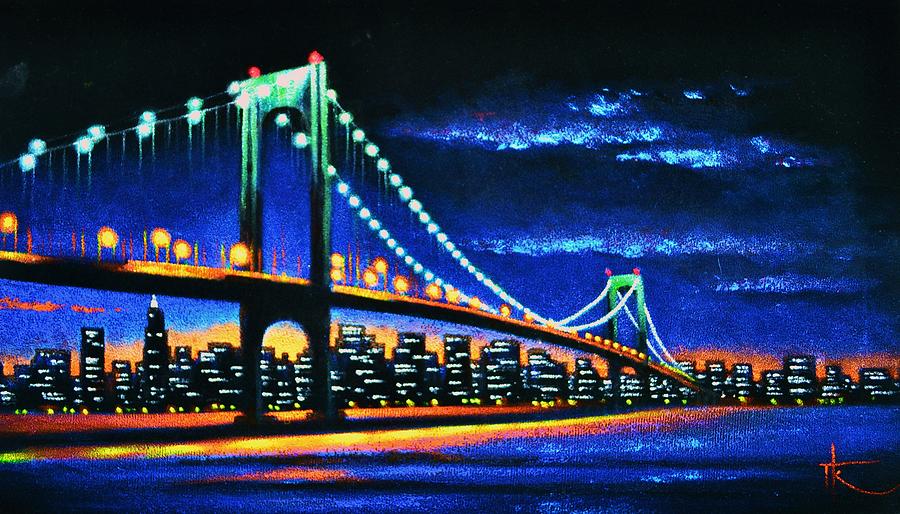This detailed painting, likely hand-drawn or digitally altered, depicts a suspension bridge spanning a body of deep blue glistening water. The bridge, adorned with white lights draping elegantly from its two large, green-painted towers, recedes from the middle left to the far right of the scene. Vibrant streaks of amber and yellow lights run along the bridge's pathway, possibly indicating illuminated streetlights. Underneath and atop the bridge, the colors shift to warm oranges and yellows, adding to the nighttime ambiance the artist aimed to capture. The bridge leads towards a distant city skyline filled with high-rise buildings, their windows glowing with countless tiny white lights. The sky is depicted in a deep dark blue, almost black at the top, transitioning to lighter blue with hints of white and yellow that suggest scattered clouds. The artist’s signature is visible in the bottom right, emphasizing the personal touch in this striking cityscape scene.